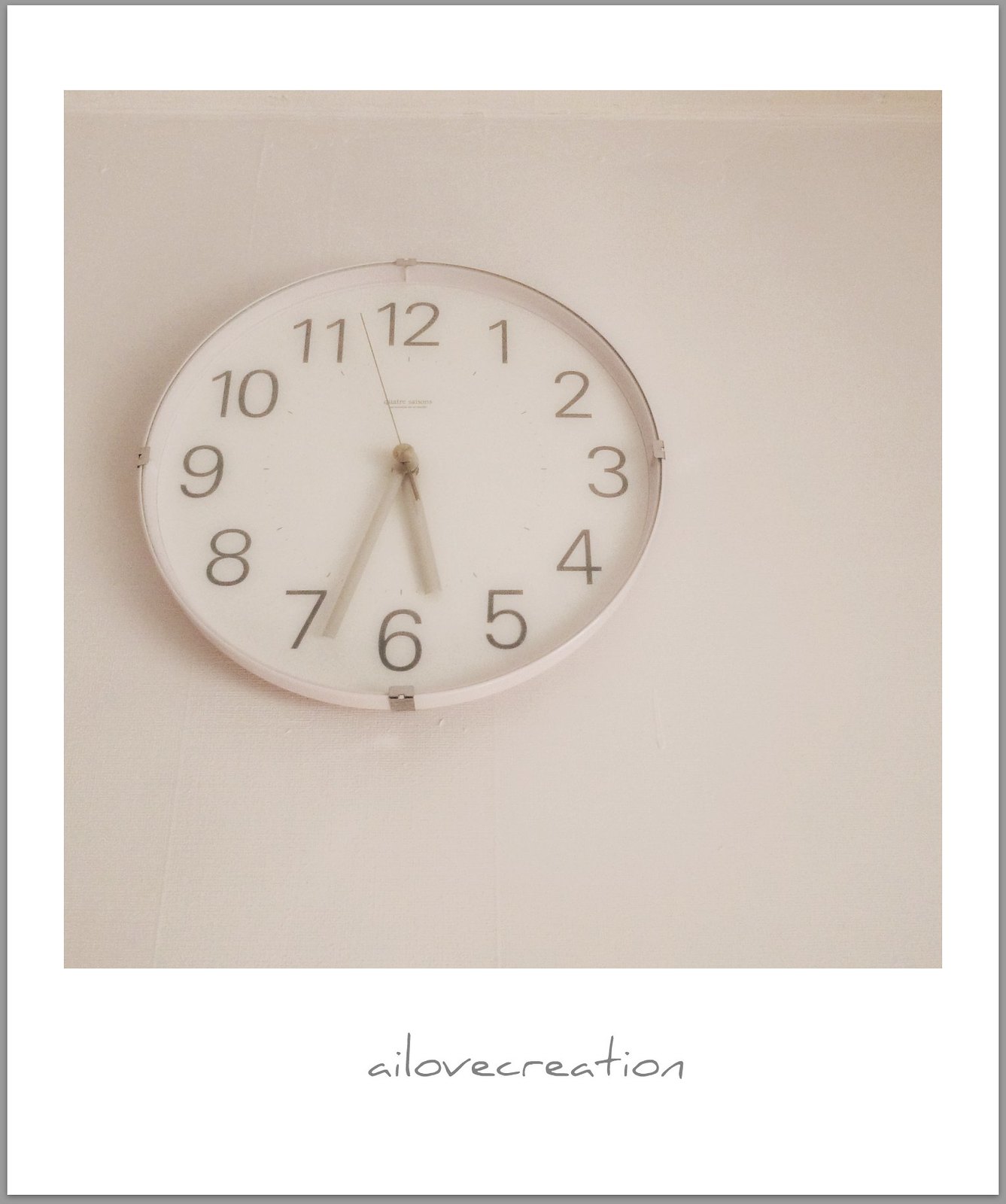A beautifully composed graphic image showcases an analog wall clock set against a pristine white or beige background. The clock features a sleek design with a white metal casing and a white face adorned with bold black numbers. Its minute and hour hands are rendered in an elegant gray, contrasted by a striking black second hand. Just beneath the 12 o'clock mark, a small brand logo subtly enhances the clock's minimalist charm. The entire image is encased within a tasteful white graphic mat, punctuated by a creative, informal font inscription in dark gray at the lower border that reads "AI Love Creation." This is further framed by a complementary dark gray border, adding a touch of sophistication to the overall presentation.